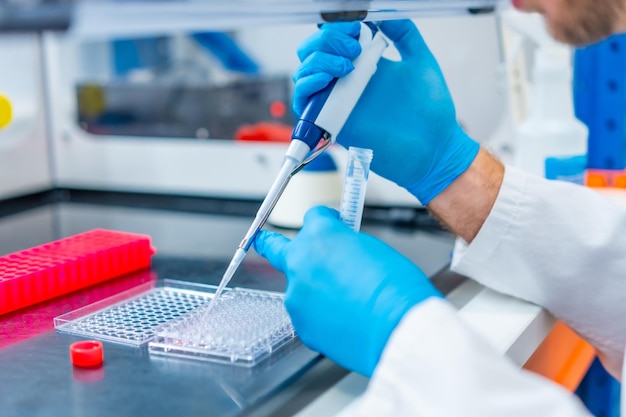In a pristine medical laboratory, a lab technician meticulously works with precision instruments. Their hands, clad in bright blue latex gloves and enveloped in the white sleeves of a lab coat, deftly handle a white and blue tool that tapers to a fine point. This instrument is poised over a tray filled with numerous tiny receptacles, suggestive of a high-throughput testing setup. The technician appears to be transferring liquid from a large vial in their left hand into these small vials or wells in the tray. A red-capped item and what looks like a round lid for the tube can be seen on the metallic work surface, along with various other lab apparatus in the background. The scene is one of careful scientific process, perhaps involving the preparation of samples or the precise dispensing of reagents into the vials.